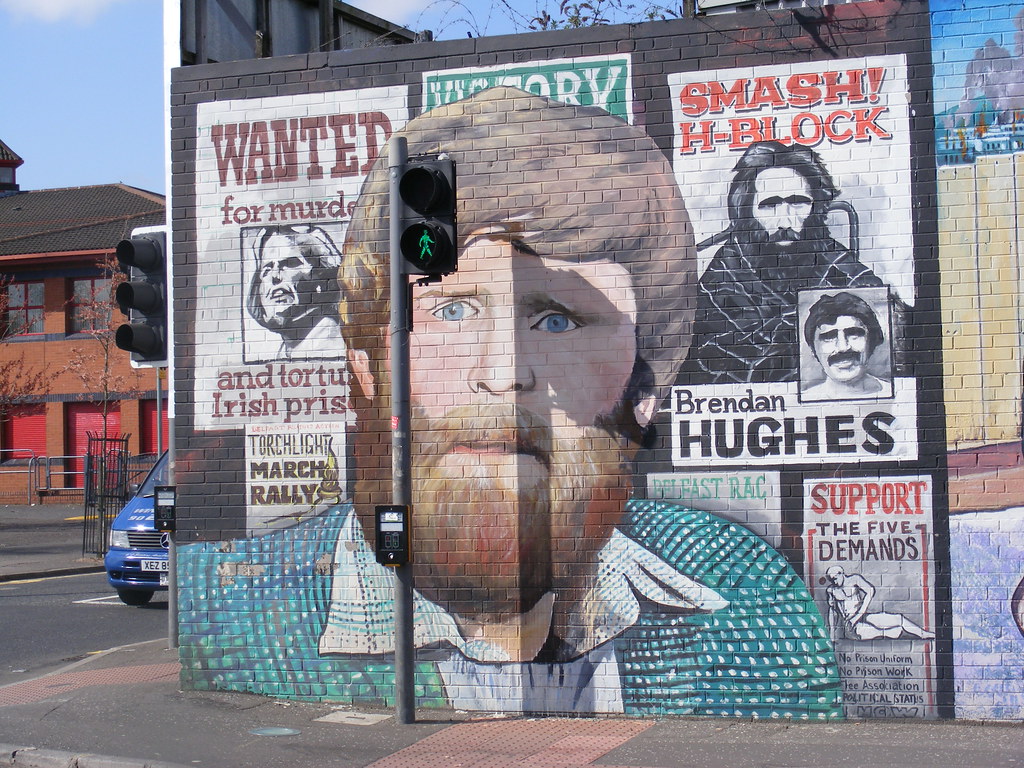In this image, a striking mural dominates a brick wall on the side of a building, depicting a large white male with bright blue eyes, a long, scruffy orange-brown beard, and full brown hair. He is adorned in a teal-colored dress shirt speckled with white dots and a white collar with blue trim. Surrounding the mural are several politically charged posters, painted on the wall, including a "Wanted for Murder" notice, a "Torchlight March Rally" announcement, and a "Smash H Block, Brendan Hughes" declaration. Another prominent sign advocates for the "Five Demands," listing grievances such as "No Prison Uniform," "No Prison Work," "C-Association," and "Political Status." In the background to the left, a brown building with red doors and trim is visible, alongside a partially seen traffic light and the front part of a blue vehicle, with cars driving on the street, hinting at the urban setting of the mural.